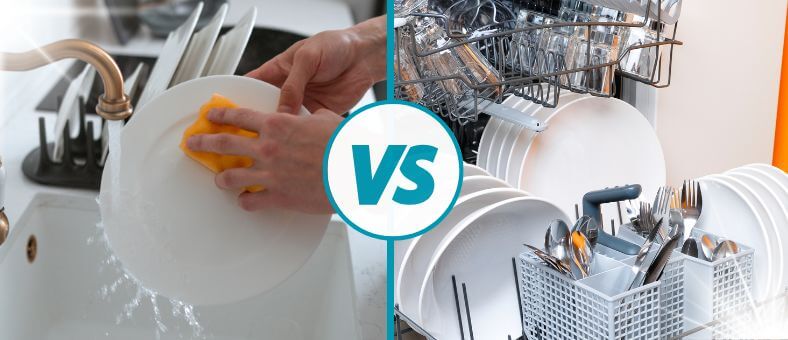The composite image illustrates a comparison between hand-washing dishes and using a dishwasher. On the left side, the photograph shows a close-up of a white person's hands scrubbing a white plate with an orange sponge under a bronze faucet, with water splashing onto the plate. Behind the active washing scene, a black dish rack holds several large and small clean plates on a white countertop beside a white sink. A turquoise line, in the middle of the image, separates this scene from the right side, with a white circle outlined in turquoise prominently displaying "VS" in the center. The right side photograph reveals the open interior of a dishwasher loaded with white plates, bowls, and various utensils including forks, spoons, and knives on the bottom rack, alongside stemmed glasses and regular cups on the top rack. The background features a white wall with bright orange highlights accentuating the clean setup. This side-by-side layout provides a clear visual distinction between the manual effort of hand washing and the convenience of using a dishwasher.